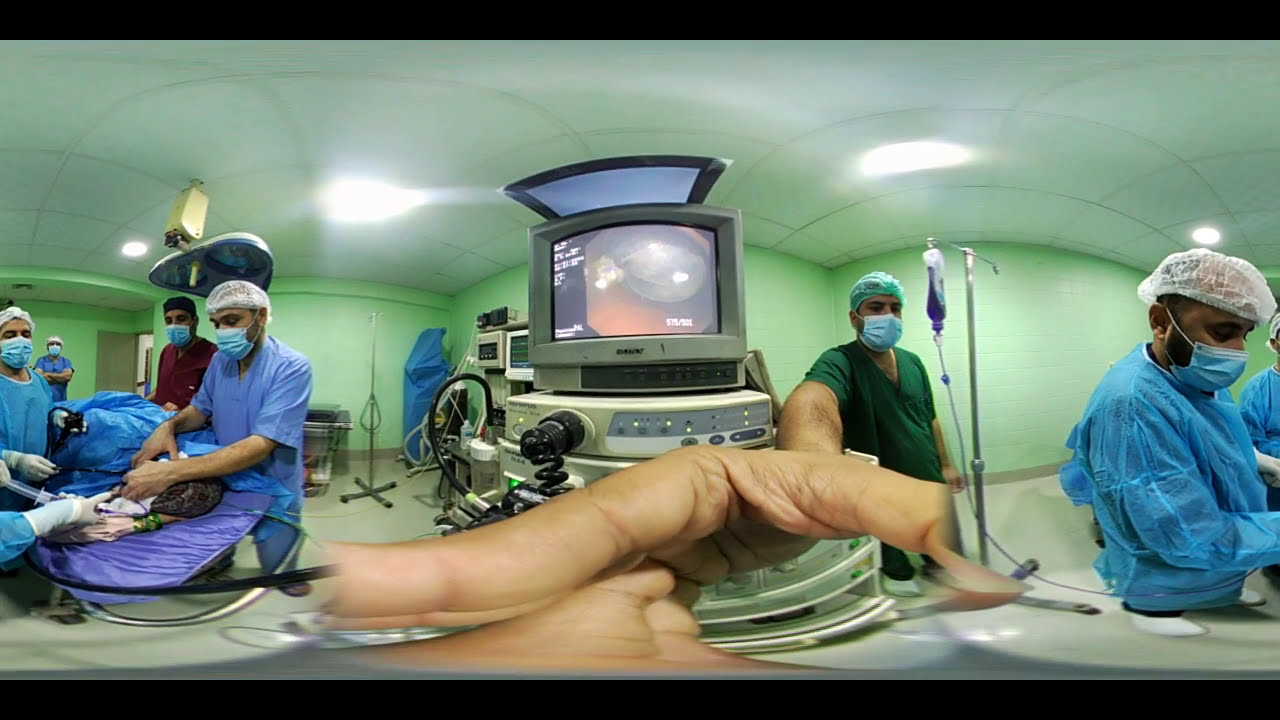The image captures a busy operating room within a medical facility, its walls painted a distinctive lime green. Central to the scene is a large piece of machinery with an attached monitor displaying internal visuals of the patient's body, presumably from a camera used during the surgery. The room is bustling with a team of medical professionals; a mix of surgeons and assistants all adorned in blue gowns, white caps, and face masks—some positioned to the left of the image around the patient, with others to the right. The ceiling is white, featuring unique curved decorative elements, and illuminated by fluorescent lights. The overall environment and arrangement of the medical staff create a sense of intense focus and meticulous care within the operating room.